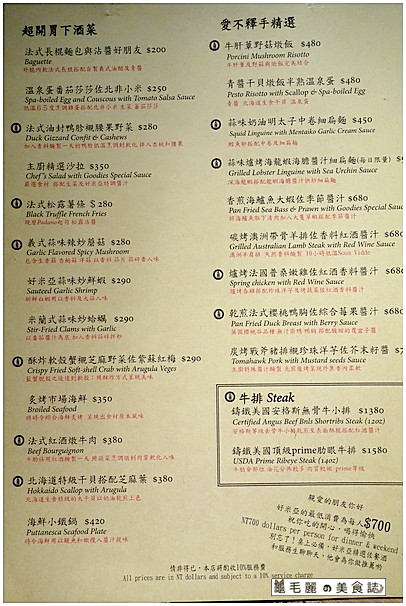This photo features a menu page with an off-white background, reflecting slight shadowing from an overhead light source. The layout is divided into two distinct columns, each topped with a darker printed heading. Predominantly written in Japanese, the menu also includes English translations for each item. Small dark circles with markings, presumably for aesthetic or organizational purposes, accompany each menu entry. At the bottom, a bold rectangle highlights "Steak and Certified Angus Beef" and "USDA Prime Rib" in large, clear lettering. Menu prices are listed in dollars. Additionally, red text under each item hints at the presence of a third language, although its contents are unclear. The bottom right corner features a white horizontal rectangle adorned with various, unidentified symbols.